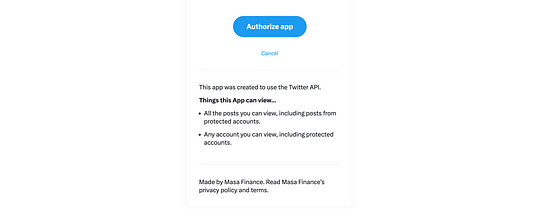The image depicts an authorization screen for an application that utilizes the Twitter API. The screen presents two options: "Authorize app" and "Cancel." The text explains that this application has been designed to access Twitter data, allowing it to view all posts that the user can see, including tweets from protected accounts. It notes that this encompasses any accounts the user can view, indicating full access to visible content, even if the accounts are protected. The app in question is developed by "Masa Finance." Additionally, the screen mentions the existence of Masa Finance's privacy policy and terms of service.